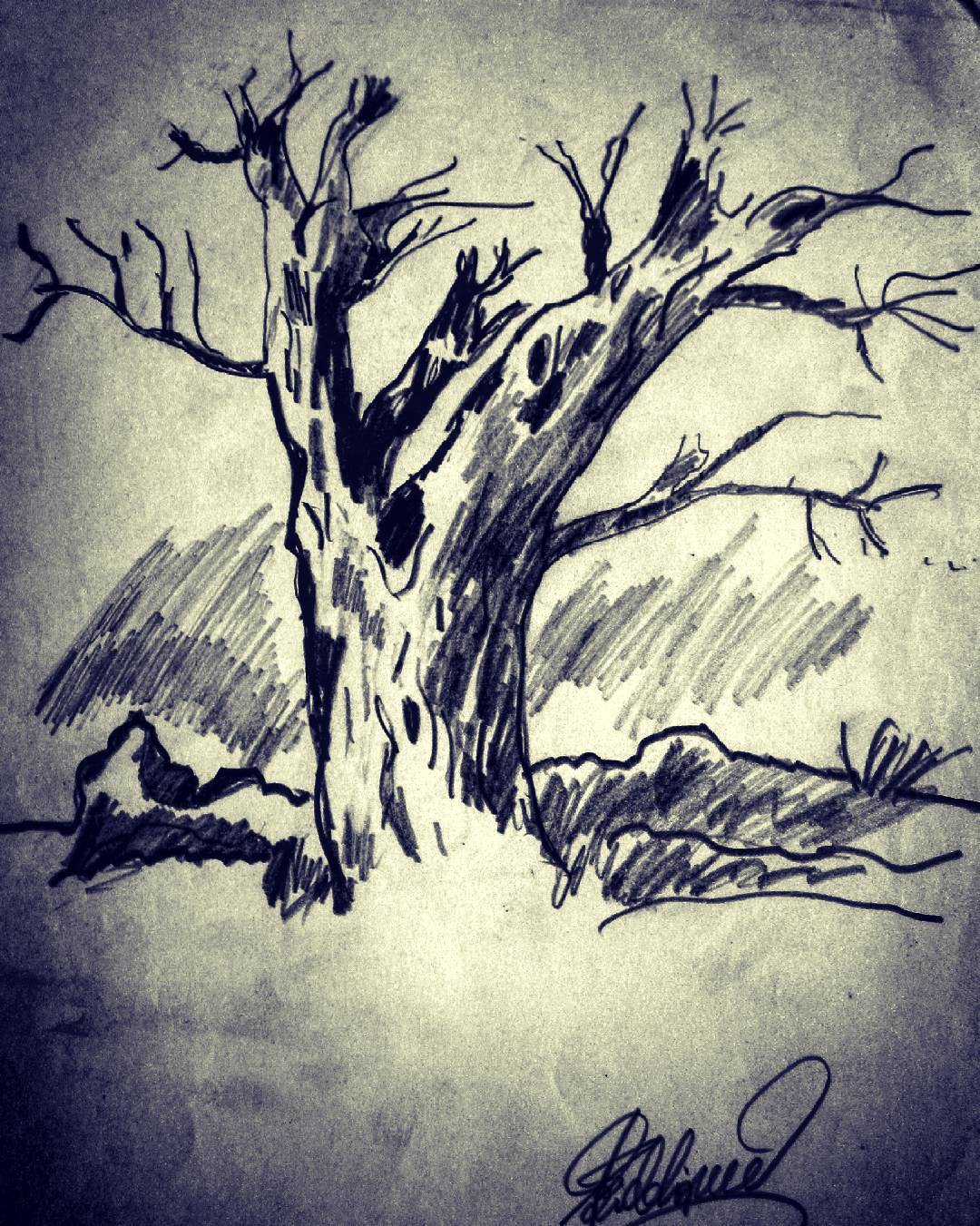This vertical, black and white drawing likely done in charcoal or ink depicts a leafless, dead tree with a large, branched trunk marked by a few holes or openings, which could serve as nests for animals like owls or squirrels. The stark, barren tree stands out prominently against a background of simple linework and shading, possibly suggesting clouds, while the surrounding ground is loosely sketched to resemble hills, shrubs, or grass. The edges of the image are darkened, creating a contrast that highlights the lighter tree. The paper itself has a yellowish beige tinge, adding a hint of warmth to the otherwise monochromatic scene. The artist's stylized and somewhat illegible signature appears in the lower right corner, beginning with the letter "R" and ending in a distinctive loop.